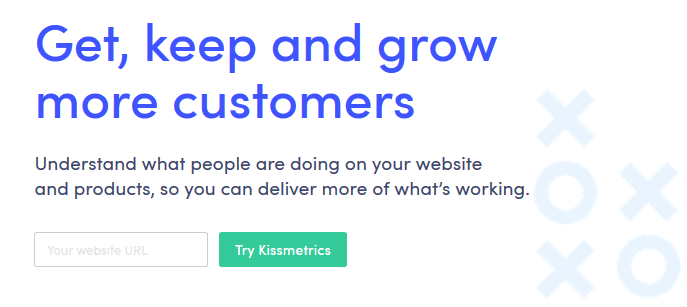The image features a visually striking call-to-action header with the phrase, "Get, Keep, and Grow More Customers," written in bold blue text at the top. Beneath this header is a white space, followed by a line of black text that reads, "Understand what people are doing on your website and products so you can deliver more of what's working." Further down, the image includes a white box on the left where users are prompted to enter 'your website URL.' To the right of this input box is a green button with white text that says, "Try KISSmetrics."

The background of the image is predominantly white, providing a clean and professional look. To the right side, there is a subtle, faded pattern of X's and O's arranged in a grid-like fashion. The sequence starts with an 'X' at the top, followed by an 'O' on the left below it, and an 'X' to its right. Below this, there is an 'X' on the left and an 'O' to its right, creating a strategically placed, almost translucent design element.